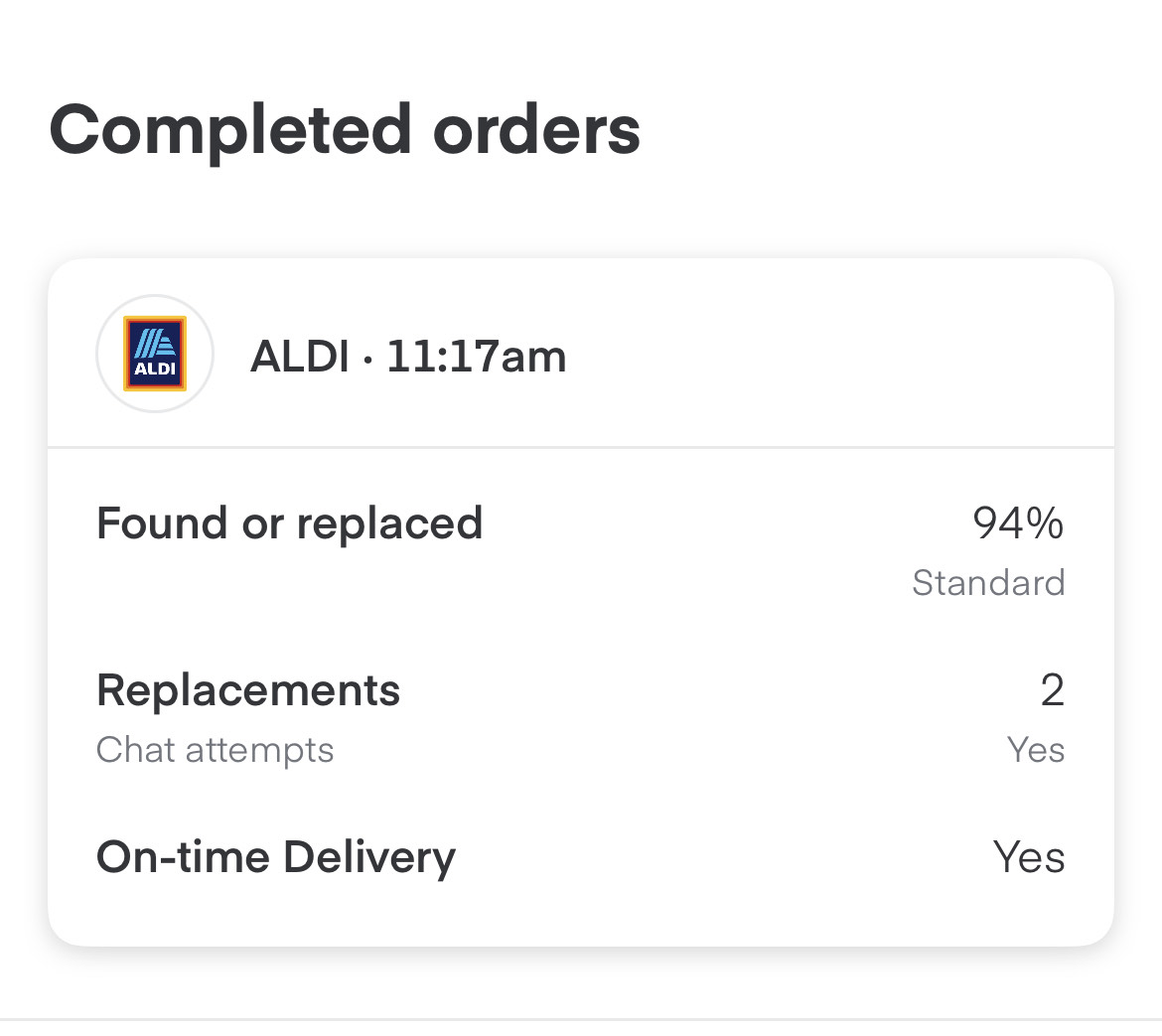This is a clean and detailed descriptive caption for the given image:

"The screenshot depicts an Aldi order update interface set against a crisp white background. Positioned in the top-left corner is the iconic Aldi logo, a blue vertical rectangle encasing a stylized teal 'A' with the word 'Aldi' written in white underneath; the rectangle is surrounded by a vivid red and yellow border. Adjacent to the logo, in bold gray font, is the heading 'Aldi 11:17 AM'. Below this, a status update reads 'Found or Replaced, 94% standard', indicating the percentage of items found or replaced in the order. The section directly beneath this is labeled 'Replacements', with 'Chat Attempts' written in lighter gray text below. To the right of these labels are succinct updates: 'To' and 'Yes', followed by 'On Time Delivery' and 'Yes'. The layout is symmetrical and user-friendly, effectively conveying essential order information at a glance. The design is straightforward, with ample empty space contributing to its clean and organized appearance, ensuring clarity and ease of interpretation for the user."